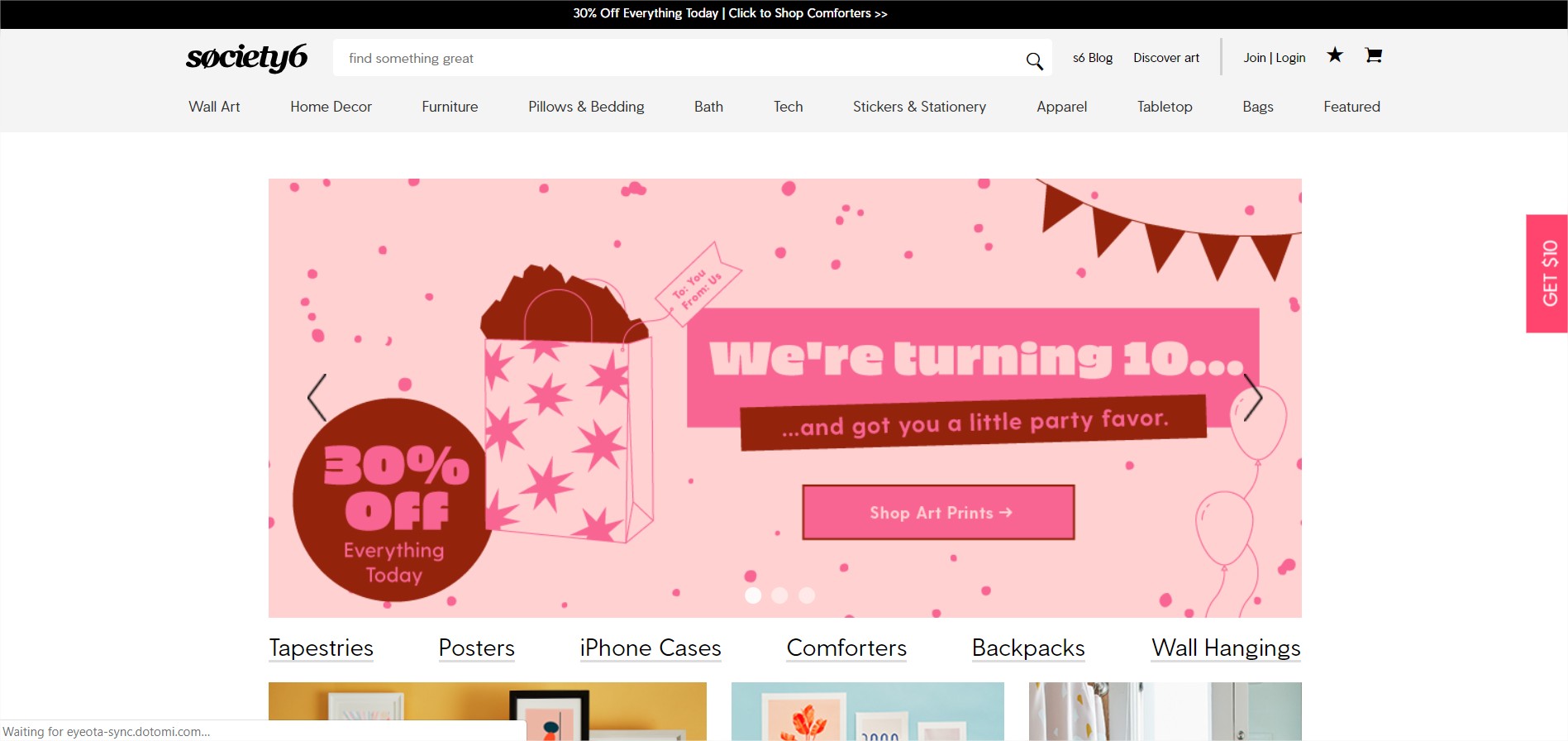A screenshot of the Society6 website captures its vibrant and celebratory design. The website's name, "Society6," is prominently displayed in sleek black lettering on the upper left-hand corner. A black navigation bar stretches horizontally across the top, featuring a convenient search bar. Below it, a gray menu bar categorizes various product offerings: Wall Art, Home Decor, Furniture, Pillows & Bedding, Bath, Tech, Stickers & Stationery, Apparel, Tabletop, Bags, and Featured items.

Centrally focused is a visually appealing banner with a light pink backdrop resembling stylish wallpaper. Adorning the center is a maroon circle with pink edges, proclaiming "30% off today" in bold, celebratory font. Beneath this, a graphic displays a pink shopping bag decorated with darker pink stars, surrounded by maroon merchandise.

Text across the banner reads, "We're turning 10..." hinting at the anniversary celebration. Festive flags appear in the upper right corner alongside the prompt to "Shop all prints." The banner continues with a playful mention, "and got you a little party favor."

Below, a partial list of featured categories includes tapestries, posters, iPhone cases, comforters, backpacks, and wall hangings. However, the images accompanying these categories are cut off, missing from the visible screenshot. The overall design is engaging, inviting users to explore the special 10th-anniversary deals and diverse product range.